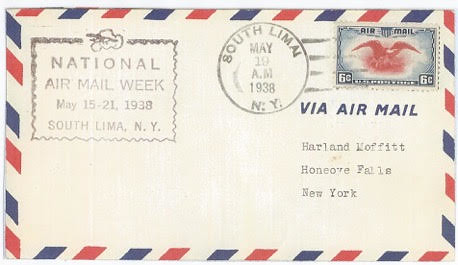This image features a scan of what appears to be an old and slightly worn envelope, likely from the past based on its off-white, dated appearance. The envelope is bordered by alternating blue and red rectangles that tilt slightly, pointing more upward on the right side and downward on the left. In the top left corner, gray stamped text reads: "National Air Mail Week, May 15 to 21, 1938, South Lima, NY." To the right of this, in the postage area, another stamp indicates: "South Lima, May 19 AM, 1938, NY." A red eagle-centered stamp, valued at 6 cents, with the words "Air Mail" on top, is also present. Below the postage area, blue text reads "Via Air Mail," and is accompanied by gray, typewritten text listing "Heartland, Moffitt, Hone, Ove, Falls, New York." The envelope is positioned slightly off-center, angled downward towards the right, offering a front-facing view that makes the details easily readable.